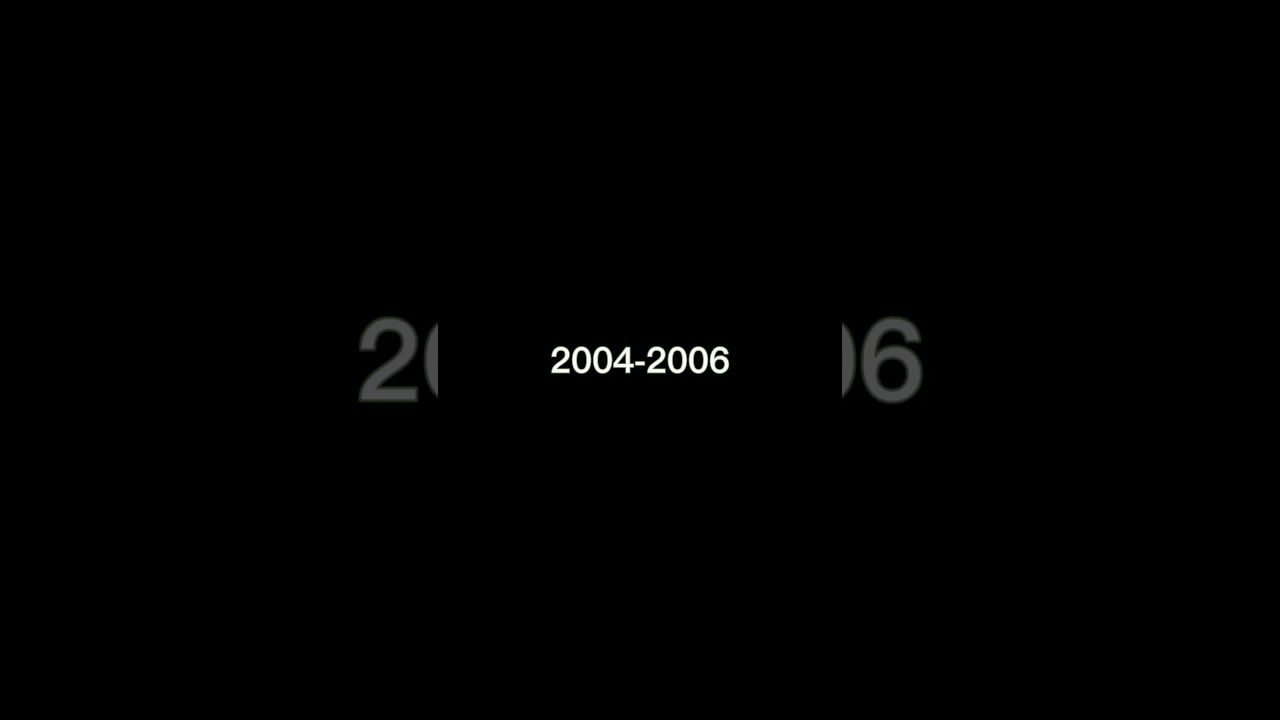The image is a horizontally oriented rectangle with a predominantly black background. It is divided roughly into three sections. At the center of the image, in a small white block font, the text "2004-2006" is clearly displayed. On either side of this central text, you can see portions of the same numbers blown up and rendered in a light gray color. On the left panel, there is a large "2" and a partial "0" just touching the edge of the central section. On the right panel, the edge of another partial "0" and a full "6" extend into the central section. The larger gray numbers seem to stretch behind the central black rectangle, suggesting a continuity of the same date range "2004-2006". This arrangement creates a minimalist and somewhat abstract visual effect, focusing solely on these specific numbers with no additional graphic elements.